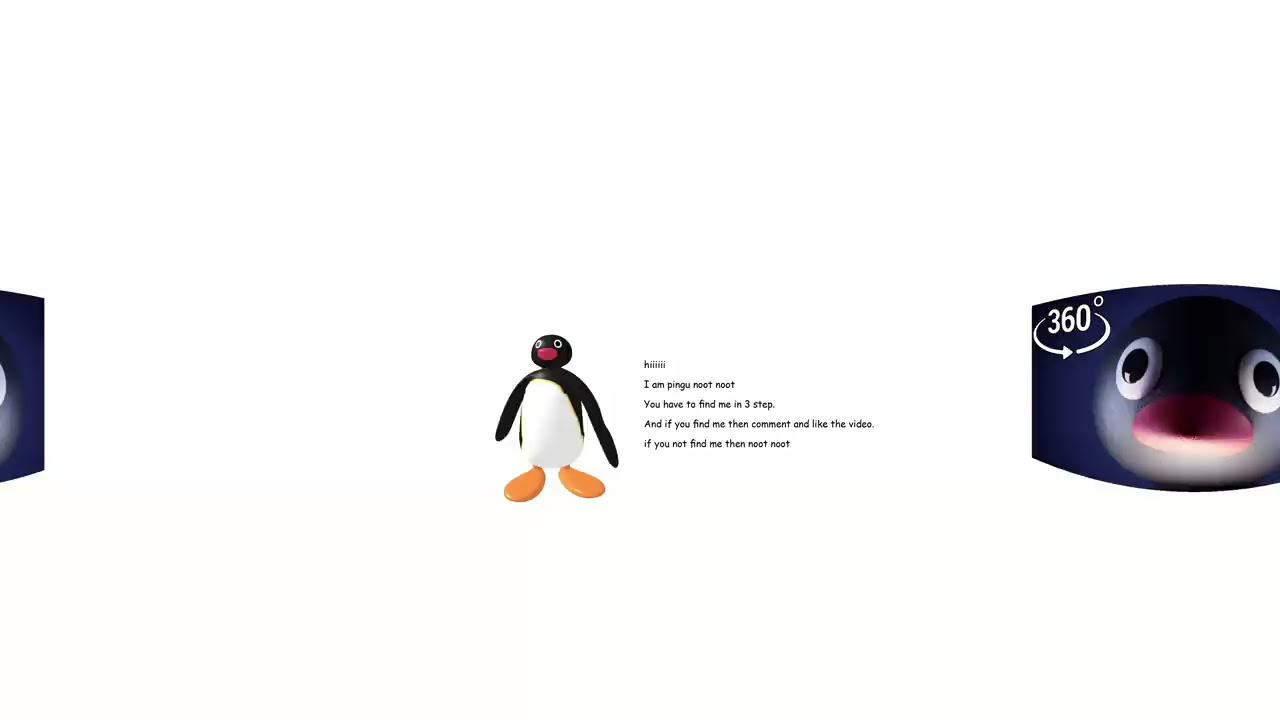This computer-generated image, set against a predominantly white background, features an off-white upper two-thirds and a pale peach and yellow gradient along the bottom third. Central to the image is a cartoonish penguin with a white belly, black flippers (one noticeably longer than the other), orange flipper feet, and an orange beak. Black eyes with white accents give the penguin a playful look. The text in lowercase black print beside the penguin reads: "Hi, I am Pingu Noot Noot. You have to find me in three steps, and if you find me, then comment and like the video. If you do not find me, then noot noot." To the left, there's a black rectangle resembling the front of a cell phone, and to the right, another black rectangle features a close-up of the penguin's head with a 360-degree logo in the upper left corner, illustrating the toy's interactive viewing capability.